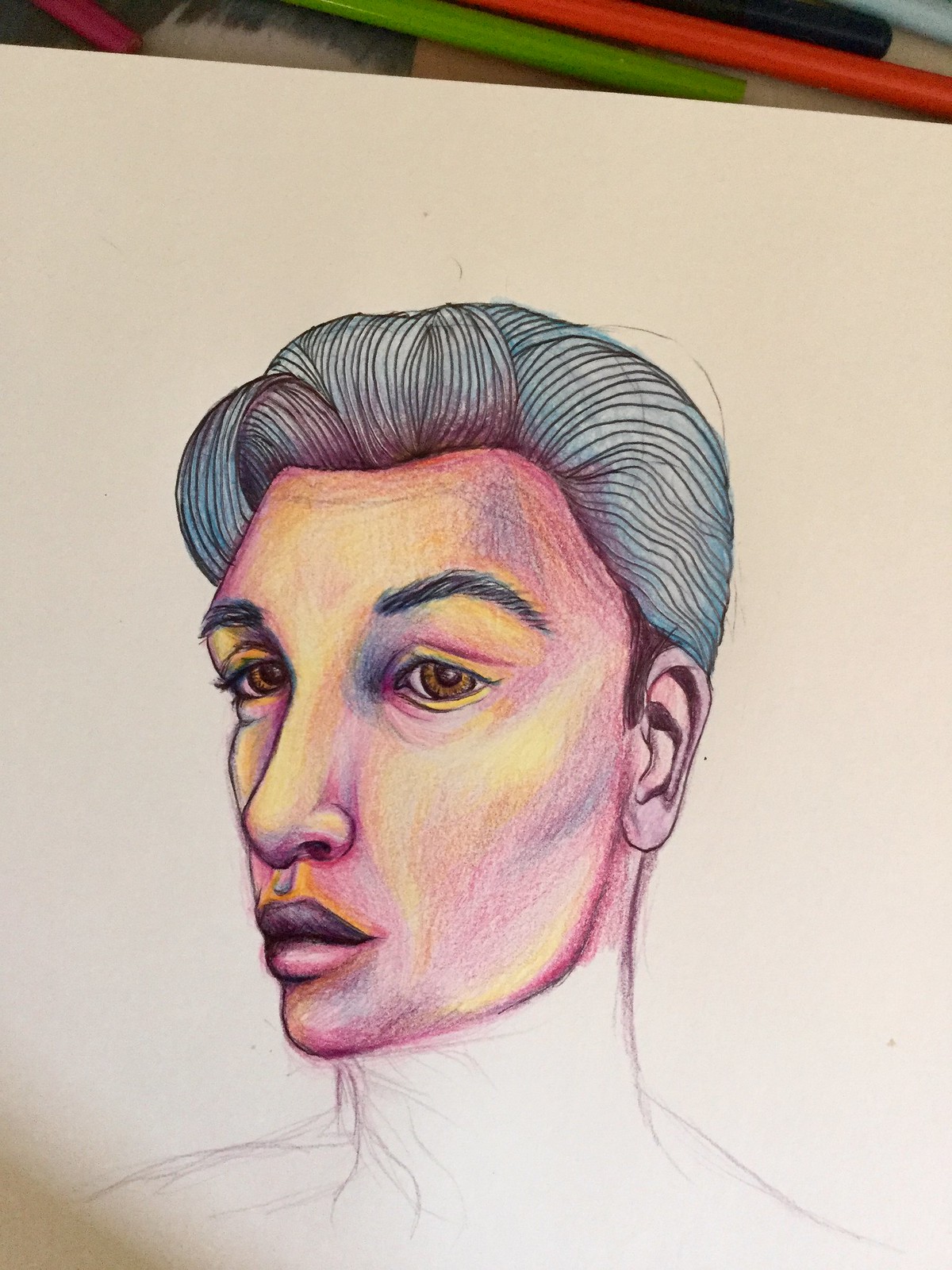The image depicts a detailed pencil drawing of a man's face and upper torso, set against a white piece of paper with colored pencils lying horizontally above it. The man has distinctive white hair combed upward, highlighted with black lines to represent strands, and an additional small black line extends from the top right. His hair has blue tints and is slicked back. He has high, arched eyebrows, and very large, slightly drooping eyes with white sclera and hazel irises. The man's long nose and wide lips are accentuated by their coloring; his lips are purple on the upper part and pink on the lower part. His face features varying shades: fair skin overall with yellow on the cheeks and forehead, and purple and pink tones on the sides and mouth area, giving it a slightly reddish hue. The body from the neck to the shoulders is outlined but uncolored, whereas the neck area is also left uncolored. His head, tilted slightly to the bottom left, adds a dynamic angle to the portrait.